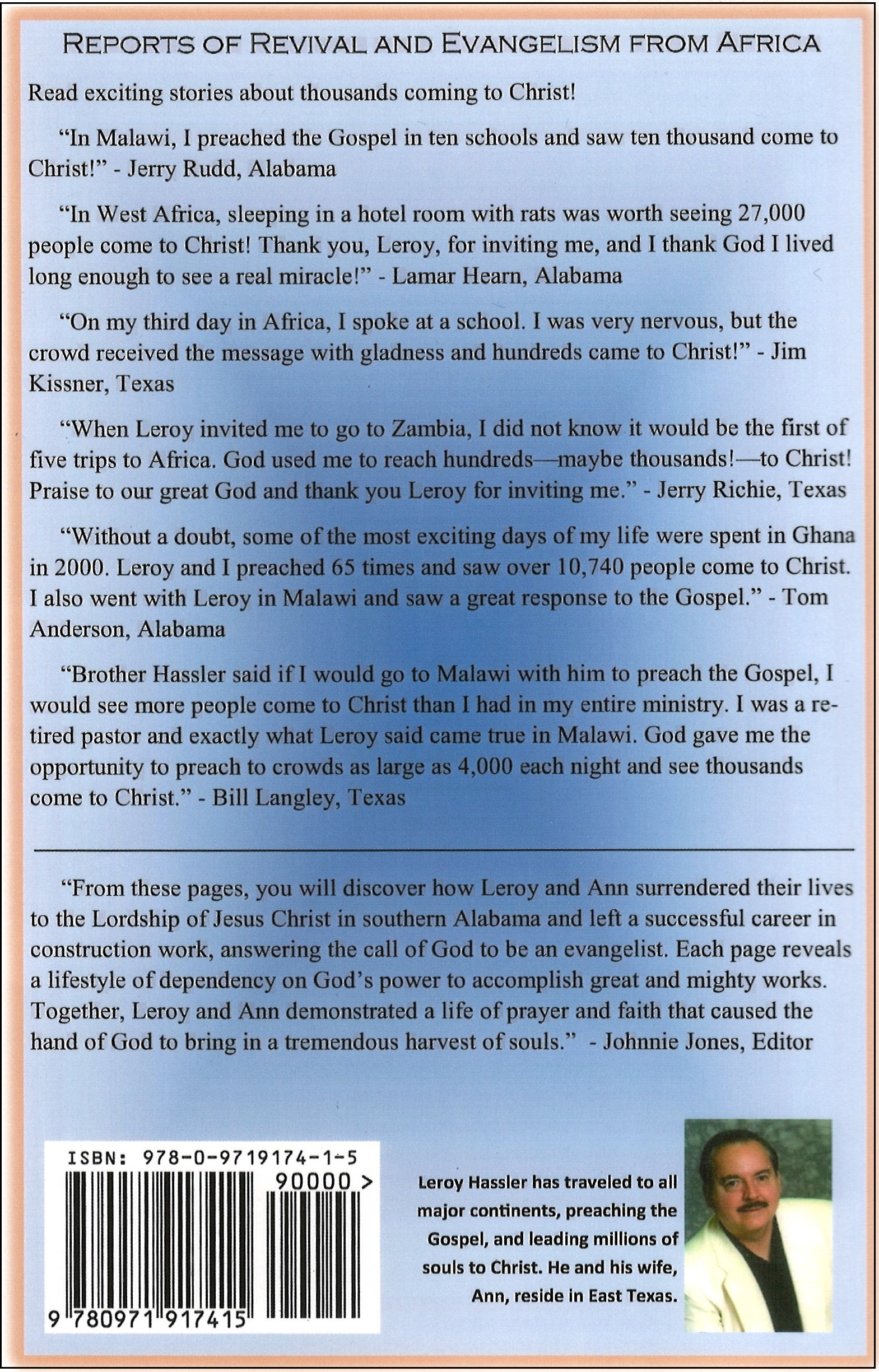The image is the back cover of a book, which is predominantly blue with a thin pink outline edging the book. At the bottom left, there is a black and white UPC barcode with numbers above and below it. To the right of the barcode, there is a small, postage-stamp-sized photo of a man who is likely the author. He is depicted wearing a white blazer over a black button-down shirt, has a mustache, dark hair, and is balding; he is set against a green background.

Adjacent to the photo, text identifies the man as Leroy Hassler, stating, "Leroy Hassler has traveled to all major continents preaching the gospel and leading millions of souls to Christ. He and his wife, Anne, reside in East Texas." Above this, at the very top of the cover, the text reads, "Reports of revival and evangelism from Africa" in black letters. Below this header, there are multiple paragraphs of text detailing the author's evangelistic efforts. One notable excerpt reads: "Read exciting stories about thousands coming to Christ. 'In Malawi, I preached the gospel in 10 schools and saw 10,000 come to Christ!' – Jerry Rudd, Alabama."

The backdrop of the cover is light blue with a faint, darker blue 'X' shape that is barely visible. Surrounding the entire text and imagery is a border that appears orange-ish beige with a thin black line on the outer edge, framing the detailed content within.